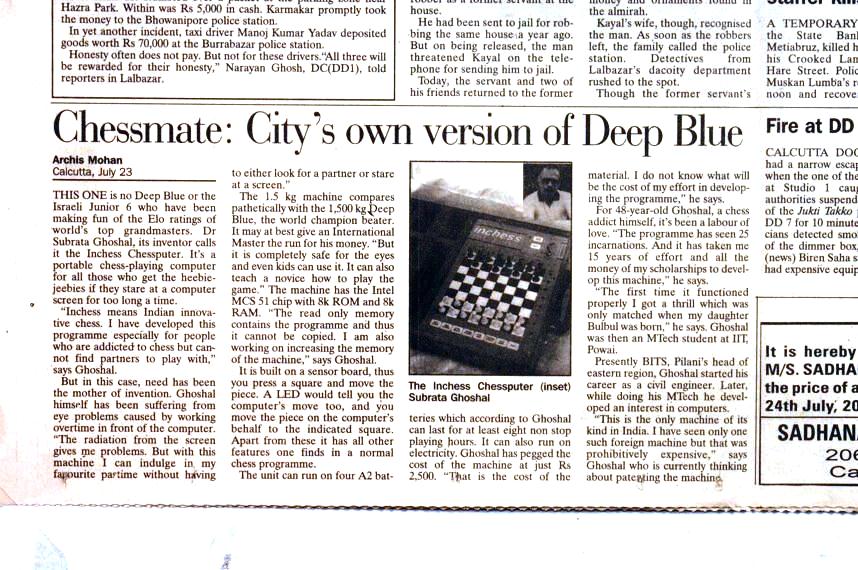The image is a clipping from a newspaper article titled "Chessmates: City's Own Version of Deep Blue." It features four neatly arranged columns under the title. The first column contains three paragraphs, while the second has two. Notably, the third column showcases a black-and-white photograph of a large chessboard, credited to Subrata Goethe, with a small portrait of a man in the upper right corner and a paragraph underneath. The final column contains four paragraphs. Written by Archie Mohan in Calcutta on July 23rd, the article discusses an innovative chess-playing computer called the "Inches Chess Putter," developed by Dr. Subrata Groshaw. This portable chess system aims to cater to chess enthusiasts, particularly those unable to find human opponents and those who face issues with prolonged screen exposure. The mention of another article on the right hints at additional topics covered in the newspaper, including a headline about a fire, partially titled "Fire at D D." The snippet ends with a fragmentary detail about the newspaper's price and the date, July 24.